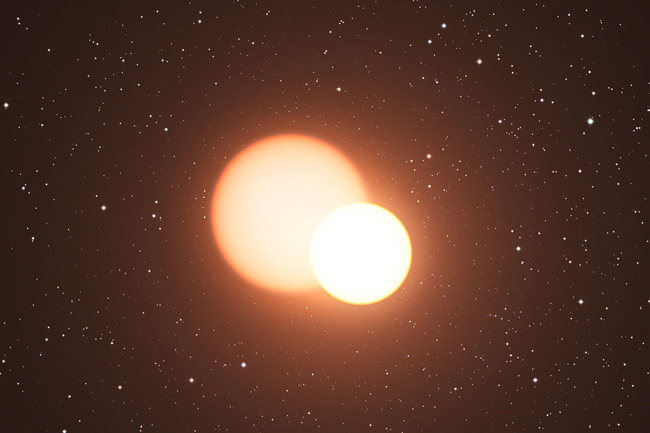This digital or AI-generated image illustrates a dramatic celestial scene resembling an eclipse. Dominating the center are two distinct, glowing orbs positioned against the backdrop of a black sky speckled with a multitude of stars varying in size and brightness. The larger orb, on the left, irradiates a diluted yellow-orange hue, with a noticeably bright orange outer edge. Slightly offset to the right and overlapping it is a smaller yet more striking vibrant yellowish-white orb, giving the impression of the start of an eclipse. The smaller orb's vibrant glow contrasts beautifully with the larger orb's softer tones. Surrounding them, the expansive dark sky is adorned with white and amber-yellow stars, emphasizing the wondrous cosmic setting.